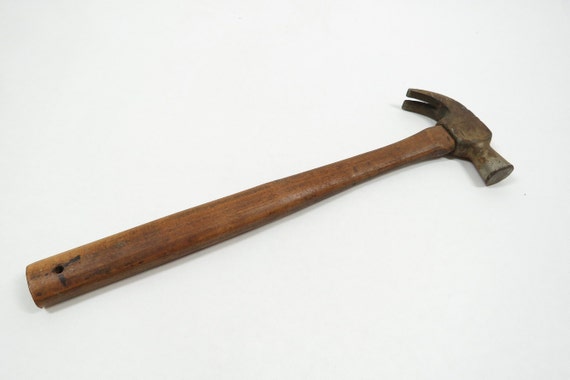This photographic image captures a singular, well-worn hammer set against a white surface. The hammer's head, predominantly made of steel, exhibits notable signs of rust, except for the tip which retains its original steel gray hue. The rust on the hammer head indicates it has been heavily used. The long wooden handle, brown with shades of black, conveys age and wear, featuring several marks and a punctured hole near its base, likely for hanging purposes. Positioned diagonally, the head of the hammer rests in the top right quarter while the handle extends towards the bottom left, making the hammer the focal point in an otherwise empty frame. The overall appearance suggests it is an old, perhaps antique, tool that has seen extensive use over time.